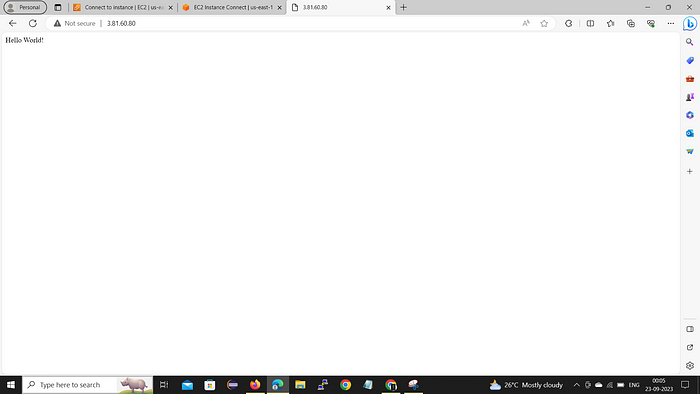A detailed caption for the described image could be:

"A cluttered Windows desktop screenshot displaying a browser window opened to a non-secure page with the URL '3.81.60.80'. The page content is sparse, displaying only 'Hello World' at the upper left corner, likely indicating a test output from a Java NetBeans application. The desktop appears to be running Windows 10 or 11 and features multiple open browser tabs, including 'Connect to Instance - FC2' and another partially obscured tab named 'interface corrected'. The taskbar at the bottom includes icons for Mail, Firefox, Internet Explorer, File Explorer, Chrome, and other applications. Additionally, a small hippo icon is visible next to the 'Type here to search' field. The desktop wallpaper or color theme isn't discernible, but the presentation suggests that this is someone's personal computer, as indicated by 'personal' in the browser tab."